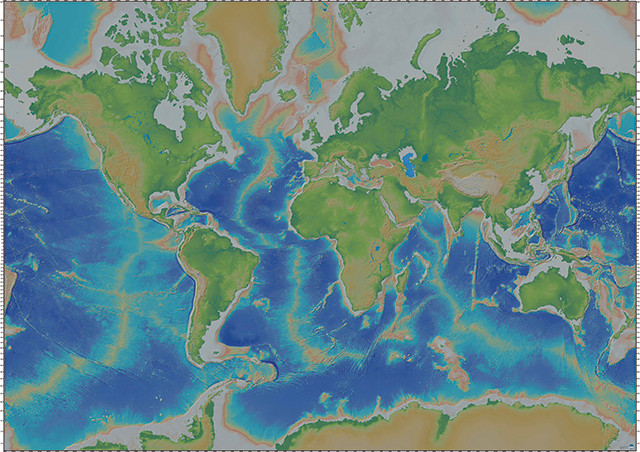This image is a flat, digital representation of a world map, showcasing the Earth's geographical features with a mix of abstract artistry. The map is characterized by distinct color variations: land masses appear in green and brown, with beige areas likely denoting desert regions, and blue tones representing the oceans and bodies of water. The blue ranges from light shades, indicating shallow waters and sandbanks, to deep, dark hues for deeper ocean areas. The Mid-Atlantic Ridge stands out in red, possibly suggesting volcanic activity or significant depth, aligning with the ridge’s geological characteristics. The top of the image is dominated by white, hinting at ice-covered regions, although there's a stark contrast with the seemingly underrepresented ice at the bottom. The map bears a resemblance to a thermal or heat map, enhanced by its digitally stylized and slightly abstract, fractal-like appearance. It features no specifying labels or text, except for barely legible markings at the bottom. The scaling along the left and right edges, along with dotted lines at the top and bottom, adds to its detailed presentation, although its exact purpose—whether topographic, thermal, or other—remains ambiguous.